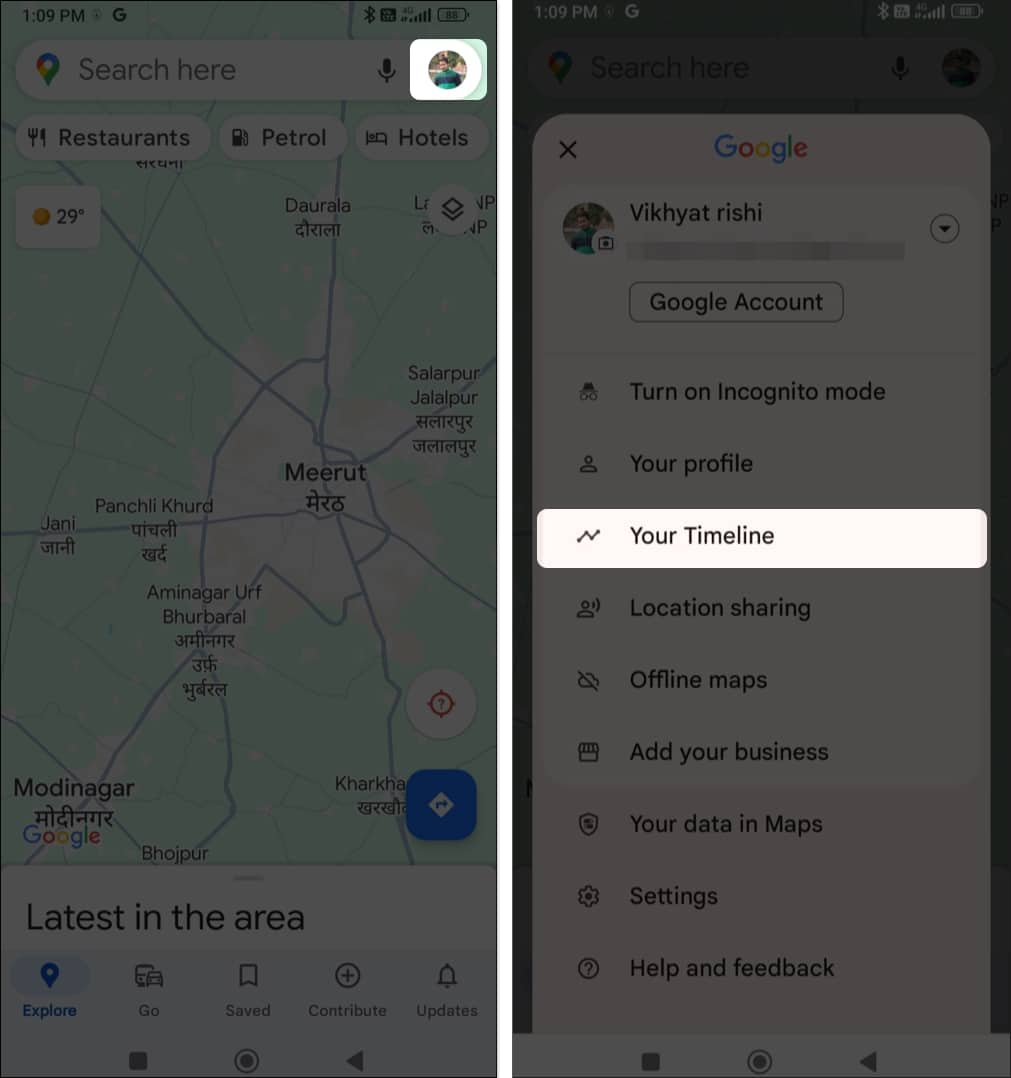This image showcases a split-screen view of two mobile device screenshots. On the left, the screen displays Google Maps with a search focused on driving directions, possibly in the city of Meerut, suggesting this could be in India. The user has selected the options for Restaurants, Petrol stations, and Hotels in the area. On the right, the screen exhibits a Google profile, specifically highlighting the "Your Timeline" option, which details the user's location history and activity.